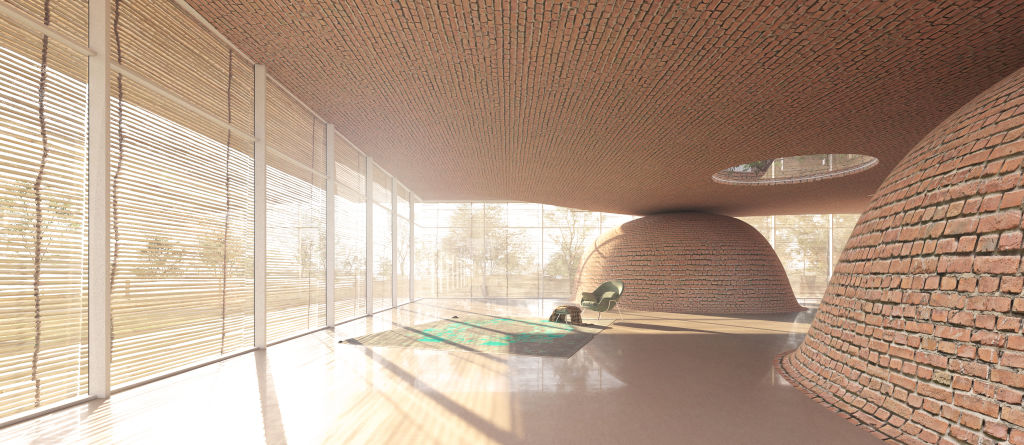The image depicts a spacious and unusually designed room, resembling an indoor patio area with prominent architectural features. Dominating the left side of the room is a large wall of tall windows, fitted with light brown, slotted shades that allow ample sunlight to stream in, creating a strong glare off the hardwood floor. Outside the windows, a view of trees can be seen. The interior floor around the central area rug—a beige rug with a light green circular pattern—appears to be epoxied wood. Positioned above the rug is a green chair.

An eye-catching feature of the room is the massive, curved mounds of red bricks that stretch from the floor to the ceiling, resembling poles but without the expected structural necessity. These brick structures are located to the right side of the room. The ceiling itself is made of light-colored brick, creating a cohesive design with the mounds. In the middle of the room, between these brick mounds, there is a notable eight-foot-wide hole or skylight in the ceiling, which appears to lead to a second floor, though there are no stairs or ladders providing access. The room is both striking and peculiar, blending elements of traditional and surreal architectural styles.